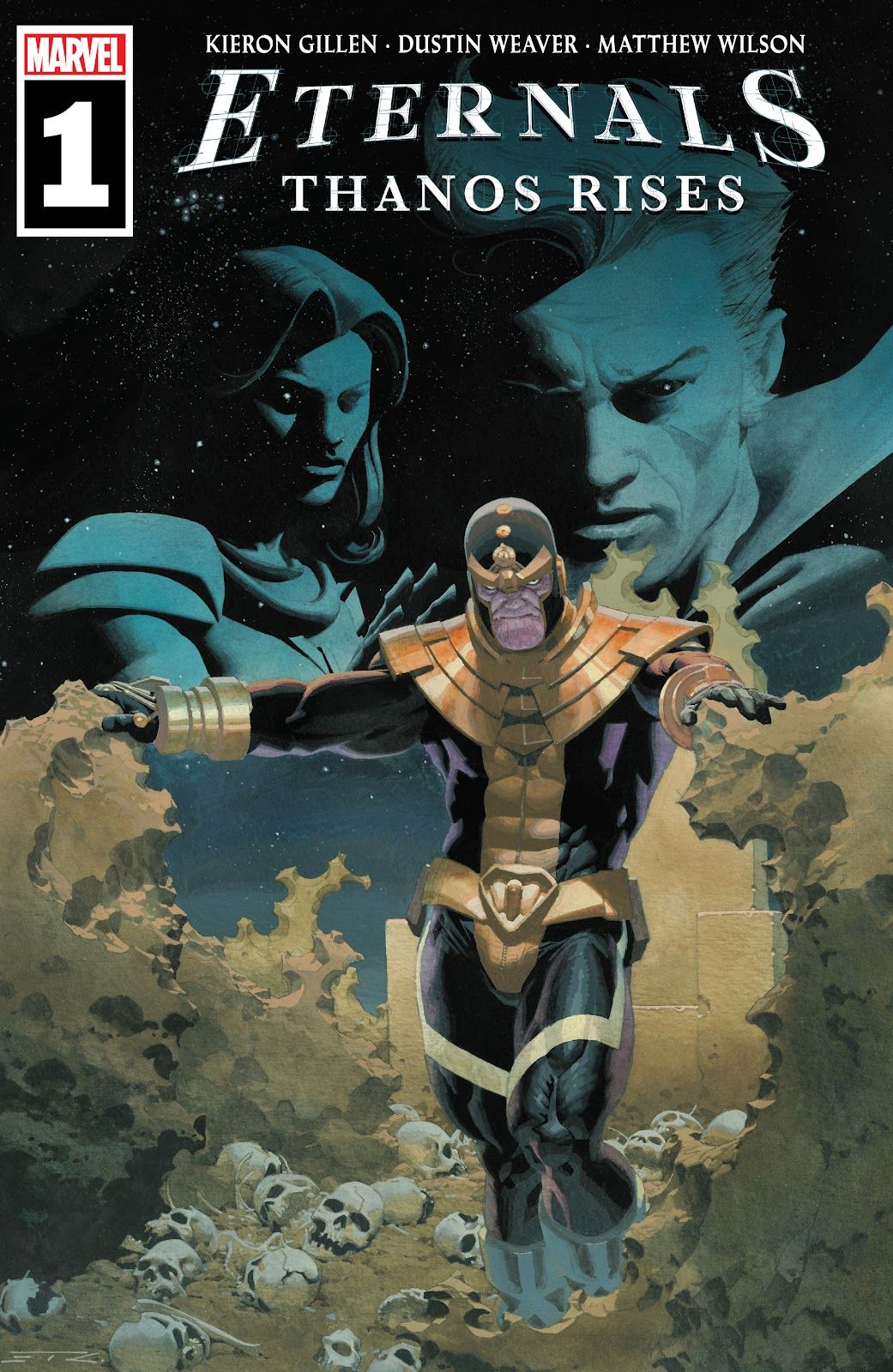This vertically-oriented, full-color comic book cover is for Marvel Series 1. Prominently displayed at the top are the names "Kieran Gillen," "Dustin Weaver," and "Matthew Wilson" in white, all-caps font against a star-studded black background. The eye-catching title, "The Eternals: Thanos Rises," arches across the top with the first "E" and final "S" enlarged to create a commanding presence. The iconic Marvel logo is situated in the corner, with "Marvel" in bold, white, all-caps text against a red background, and a bold white "1" on a black backdrop just below it.

The central figure is Thanos, instantly recognizable with his muscular build and menacing scowl. He wears a black and gold armored suit, a gold neck piece extending down his chest, and gold cuffs around his arms. In a striking pose, Thanos stands amidst a pile of skulls on a beige dirt floor, his arms outstretched to rest on two beige rocks. Above and behind Thanos hover two ghostly, blue-tinged figures. The left figure, resembling a woman with shoulder pads and a necklace, and the right, a man with a distinctive swoopy hairstyle and a collar, both peer down with an ominous air. Together, these elements create a powerful and haunting cover that draws the reader into the mysterious and dark world of "The Eternals: Thanos Rises."